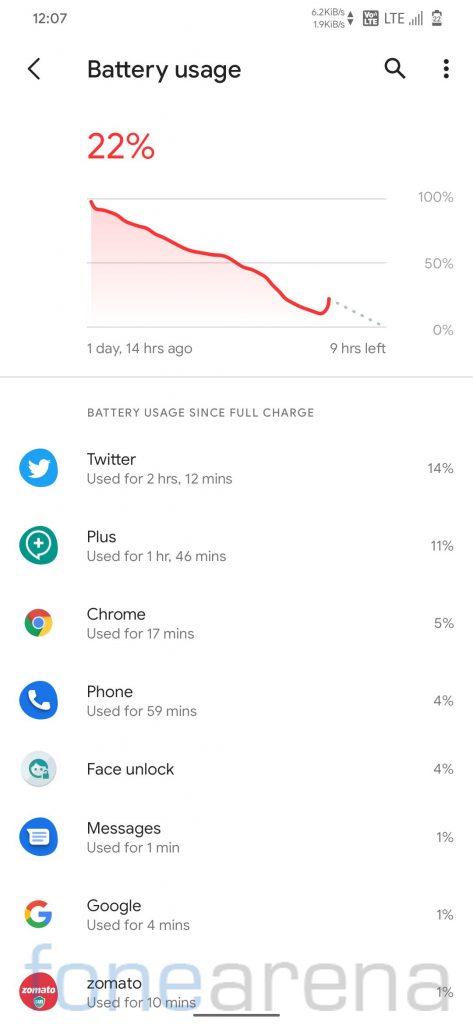This image displays the battery usage screen of an Android smartphone. The top of the screen shows the time as 12:07 PM, with the device connected to a 4G LTE network and a battery level of 22%. A battery usage graph illustrates a steady decline in battery level over a period of one day and 14 hours, with nine hours of battery life remaining. 

Below the graph, a detailed list outlines the battery consumption by various apps since the last full charge:
- Twitter: 14%, used for 2 hours and 12 minutes.
- Plus: used for 1 hour and 46 minutes.
- Chrome: used for 17 minutes.
- Phone: 4%, used for 59 minutes.
- Face Unlock: 4%.
- Messages: 1%, used for 1 minute.
- Google: used for 4 minutes.
- Zomato: 1%, used for 10 minutes.

This screen provides an overview of how the battery is being consumed by various apps over time, helping the user manage their battery usage efficiently. At the very bottom of the screen, there is a watermark for FoneArena, spelled F-O-N-E-A-R-E-N-A.